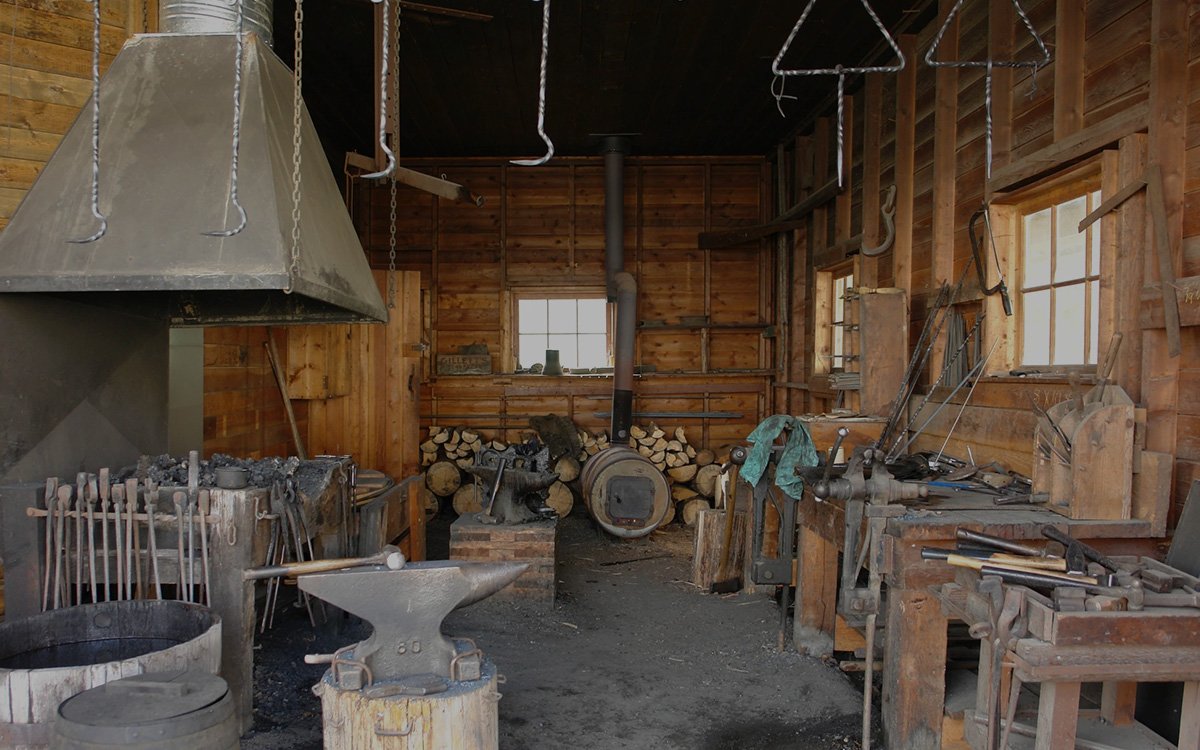The photograph captures the interior of a rustic, perhaps an ironsmith's or blacksmith’s workshop, housed in a log cabin-like structure. The walls are constructed from dark wooden slats running horizontally, with visible vertical support beams. The room is spacious and open, characterized by a tall ceiling. The floor appears blackish-gray, likely covered in ash.

In the foreground, a sturdy tree trunk serves as a makeshift table, upon which rests a large black anvil holding a hammer on its side. To the left of this setup is a stone fire pit filled with ash or coal, surrounded by small metal tools, with a large vent cover hanging from the ceiling above. Glimpsed alongside is a bucket of water.

The right side of the image showcases a wooden workbench cluttered with various hammers and tools, as well as multiple desks lined up against the wall, which also feature vices and assorted instruments. The workshop is well-lit by natural light streaming through one window on the back wall and two open windows on the right wall, casting a grayish hue over the scene.

Hanging from the ceiling on chains are about six metal hooks of various types, adding to the authentic feel of the workshop. In the background, there is another anvil and hammer on a similar tree trunk table, a round fireplace with a stovepipe and a stack of firewood against the wall. A cabinet is also tucked in the back, enhancing the workshop's functionality and lived-in appearance.